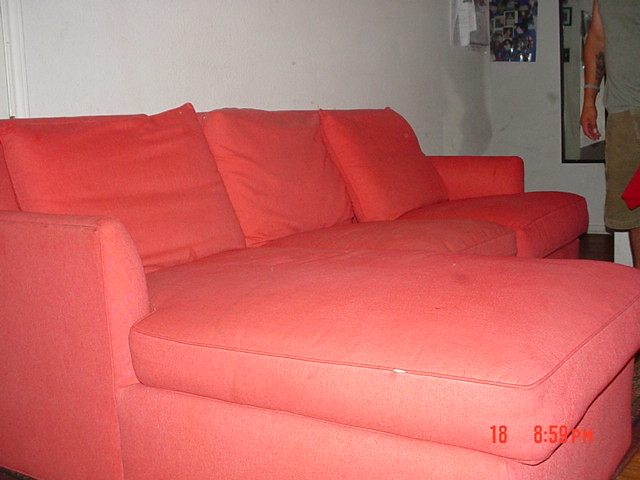This photograph captures a red sectional couch positioned in a living room against a largely undecorated white wall. The couch features a distinct section that extends outward as a footrest, making it a comfortable spot for reclining. The back of the couch faces the left side of the frame, while the footrest portion is closer to the viewer. On the wall above the couch, a mirror and a photo collage are visible. In the upper right corner of the image, part of a man can be seen. He is standing and wearing khaki green shorts and a gray sleeveless shirt, cut off at the shoulders, with a tattoo on his right forearm and a bracelet. The man's head and most of his body are cut off by the edge of the photo. In the lower right corner, there is a time stamp reading "18 8:59 p.m." in red letters. The white wall appears uneven in color, with patches that look grayer as if poorly painted.